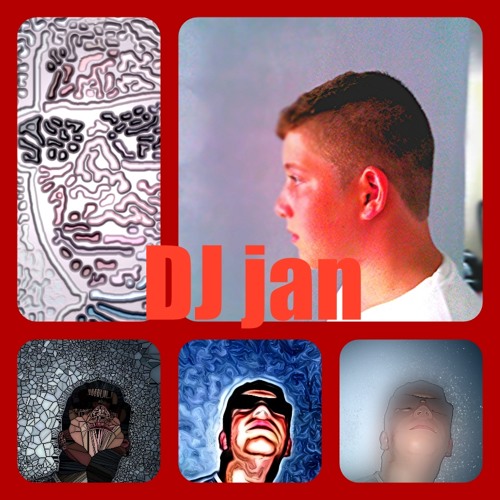The image is a vibrant, multi-layered collage primarily dominated by the colors red, purple, black, white, pink, blue, and gray. At the top right, there is a clear and striking photograph of a man with a buzz cut on the sides and thicker hair on top, wearing a white t-shirt, and gazing to the left. To the left of this photograph is a more abstract, stylized close-up of a face, possibly adorned with sunglasses, transformed into a complex texture through the application of filters. Directly below these are three distinct artistic renderings of what appears to be the same man from the top right photo. The first rendition, located at the bottom left, mimics a stained glass appearance, giving the image a broken yet vibrant look. Next to it on the right, the second version highlights a wavy, oil painting-like effect. The last depiction on the bottom right features a soft, foggy filter with a glowing outline around the man. The collage features 'DJ JIN' in red lettering centrally located within the composition, implying an artistic graphic designed for social media sharing. The objects within the image are well-positioned, maintaining individual spaces without overlapping, contributing to a clean and organized aesthetic.